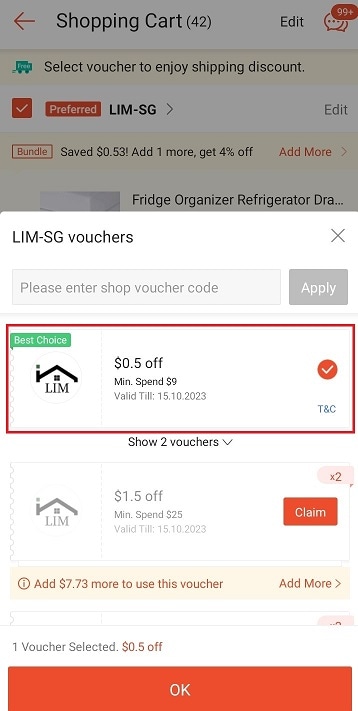Upon first glance, this web page appears to be a bustling e-commerce site. A user currently has 42 items in their shopping cart, which is prominently displayed. There are various notifications, exceeding 99 in number, indicating potential updates or alerts.

Highlighted is a prompt urging the user to "Select a voucher to enjoy a shopping discount." The system suggests that by selecting the preferred LIMSG edit bundle, the user can save 53 cents. Additionally, it advises that adding one more item to the cart will grant a 4% discount.

The "Bridge Organizer" and other LIMSG vouchers are also brought to the user's attention. Specifically, there is an option to enter a shop voucher code to get either 50 cents or 5 cents off, with a minimum spend of $9 and valid until October 15, 2023. Another set of vouchers offers discounts of $1 or $1.50 off for a minimum spend of $25, also valid until October 15, 2023.

To utilize these vouchers, the user should add $7.73 or more to their cart. Once a voucher is selected, the user can confirm by clicking "OK." 

Overall, the page is filled with various options and promotions designed to maximize savings while encouraging additional purchases.